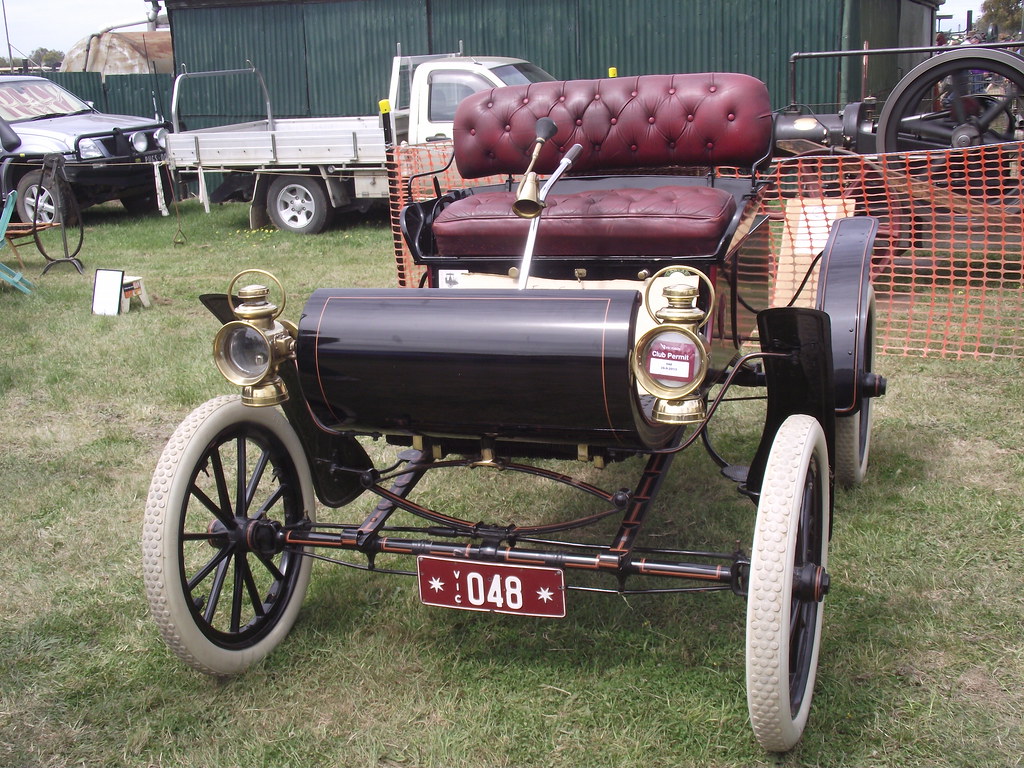The image depicts a scene behind a dark green garage-like building, possibly in the yard of a construction site or a car dealership. In the foreground stands a vintage, early 1900s automobile with a burgundy-red leather seat and no body covering, giving it the appearance of a sled on wheels. The car features small, white tires resembling those of a bicycle, and it has a front license plate reading "VIC 048" in white text with a star on either side, set against a burgundy background. The car is equipped with two small headlights and a horn, enhancing its old-fashioned charm. Situated on a grassy field, the vintage car is accompanied by an assortment of old cars, including a white car and an old white pickup truck, as well as various equipment in the distant background.